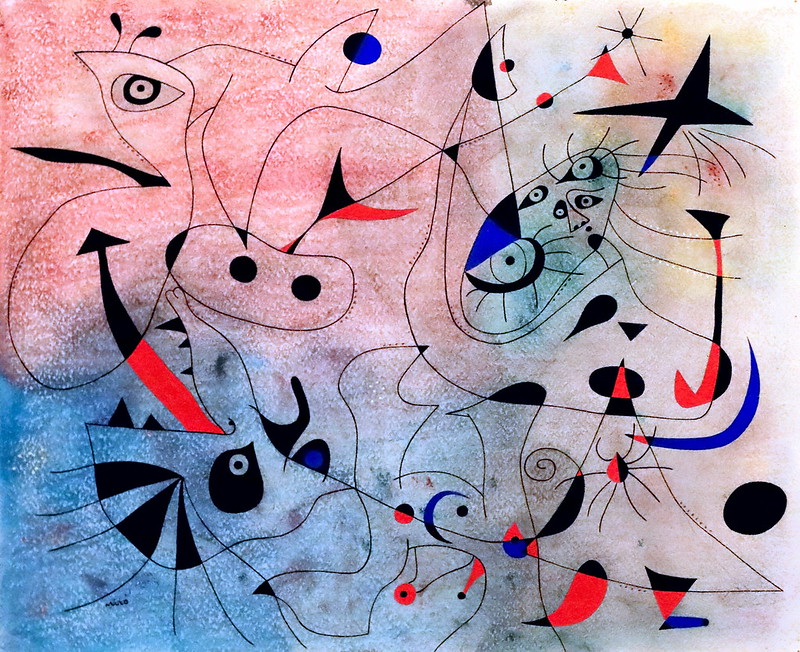This is a detailed, horizontal, rectangular modern art painting, rich in abstract elements and vibrant colors. The background landscape transitions through a spectrum, starting with a deep blue in the lower left corner, blending into gray and then pink in the top left, which gradually fades into gray and descends into the blue on the right side. The canvas is intertwined with numerous thin black lines connecting various shapes and figures. 

Prominently, there are whimsical forms hinting at animals: a fish hook, a fish, an oval with eyes and a tail, a star shape, and a spider. Some of these figures feature eyes and tails, and there's a depiction of bugs. On closer inspection, the top with a pink background suggests an abstract pig, noticeable by its eye and nostrils, while the light blue bottom left resembles a lizard with a red tongue and an arrow-like tail. The right third of the artwork, set against a lighter backdrop with touches of white and yellow, contains swirling reds, royal blues, and sporadic black circles and triangles.

Overall, the painting is a mesmerizing blend of colors and shapes, depicting a chaotic, yet captivating collection of abstract animal forms linked by expressive black lines.